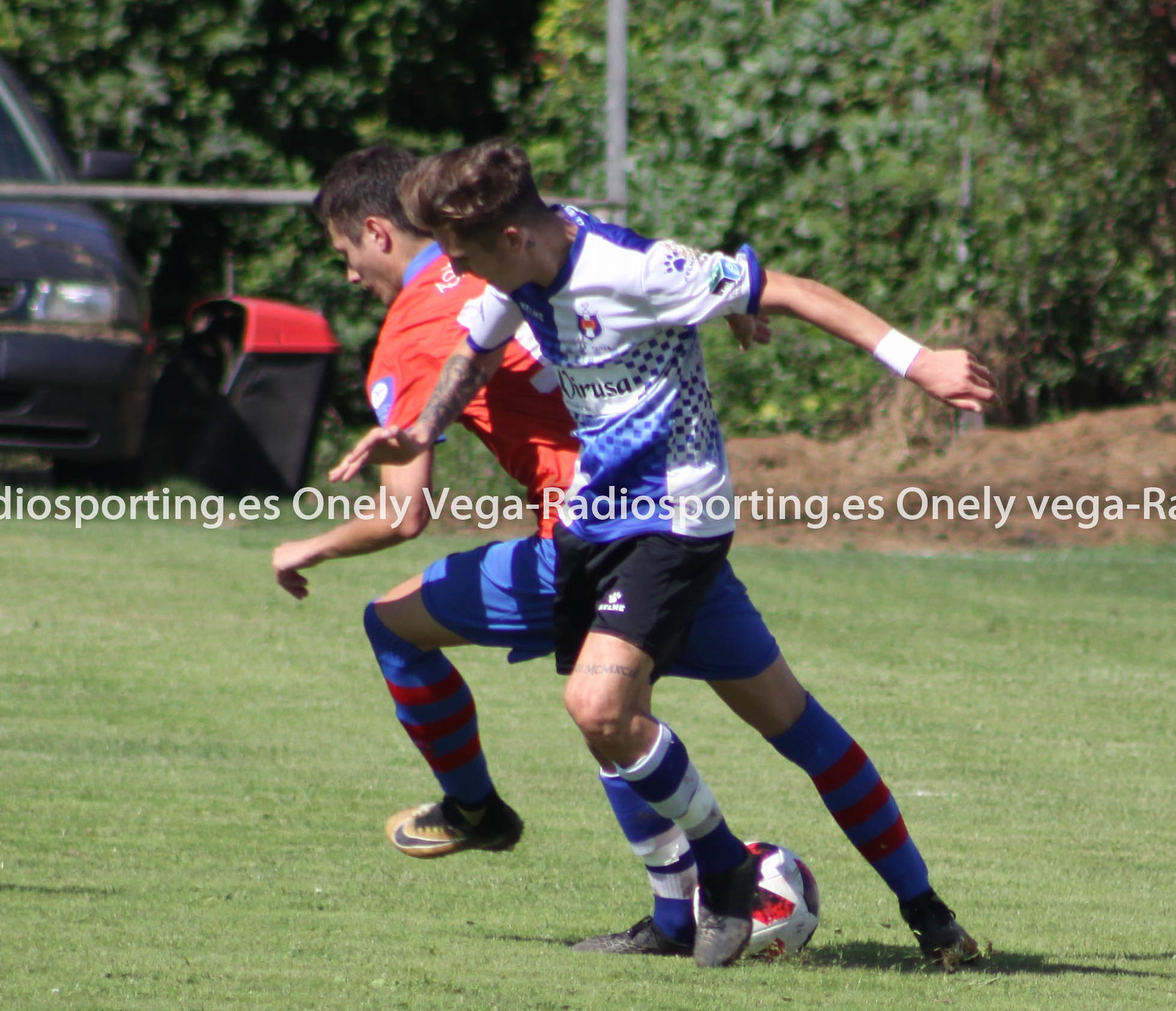In this square image taken with a camera, likely an iPhone, two young soccer players around 20 years old are captured mid-collision as they strive to control a soccer ball. The foreground features the players and the ball, while the background is split between a green field of grass and a line of trees and foliage. A black car is partially visible in the upper left-hand corner of the image. 

The player closer to the camera is wearing a blue and white short-sleeved jersey that partially reads "Verusa," black shorts, and blue and white striped socks paired with black cleats. He has brown hair and a tattoo on one forearm. The second player, seen more from the back and side, sports a red and blue jersey with an unreadable white number on it, blue shorts, and blue and red socks matched with white cleats featuring a blue Nike logo. 

The soccer ball, located between their feet, is white with red and black markings. The image also contains overlaid text including partial website URLs such as "onlyvega-radiosporting.es," repeated in various forms across the photo.